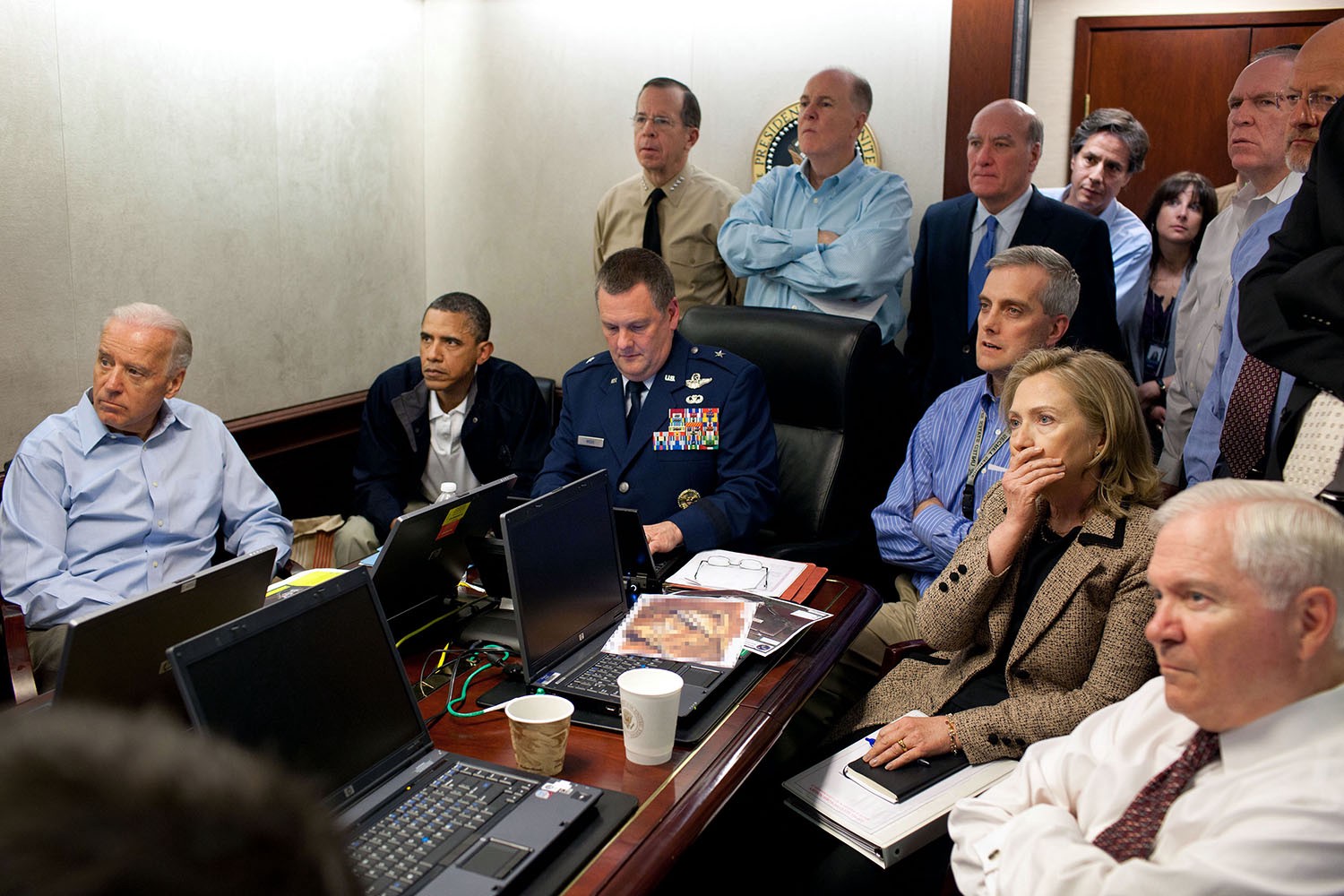In this historical photograph captured in the Situation Room, various prominent government figures react with intense focus and concern while watching an event unfolding off-camera to the left. At the dark brown table with a gold inset border, five laptops are positioned, one of which has a blurred-out image on its screen. Centrally seated from left to right are key figures: Joe Biden in a blue shirt, his white hair distinguishing him, and Barack Obama in a black coat and white shirt who is leaning forward in his chair. Both are closely watching, alongside a military general adorned with medals and a black tie, seated in a plush black leather chair. To the general's right is a man in a blue striped shirt, followed by Hillary Clinton, her light blonde hair styled with a part to the left. Clinton, wearing a brown tweed jacket over a black shirt, appears particularly concerned, her right hand covering her mouth in a gesture of shock and her other hand resting on a file folder. The room, likely the Situation Room, features additional, unidentified individuals in the background, bringing the total to approximately fifteen people, most of whom share a grave and attentive demeanor.